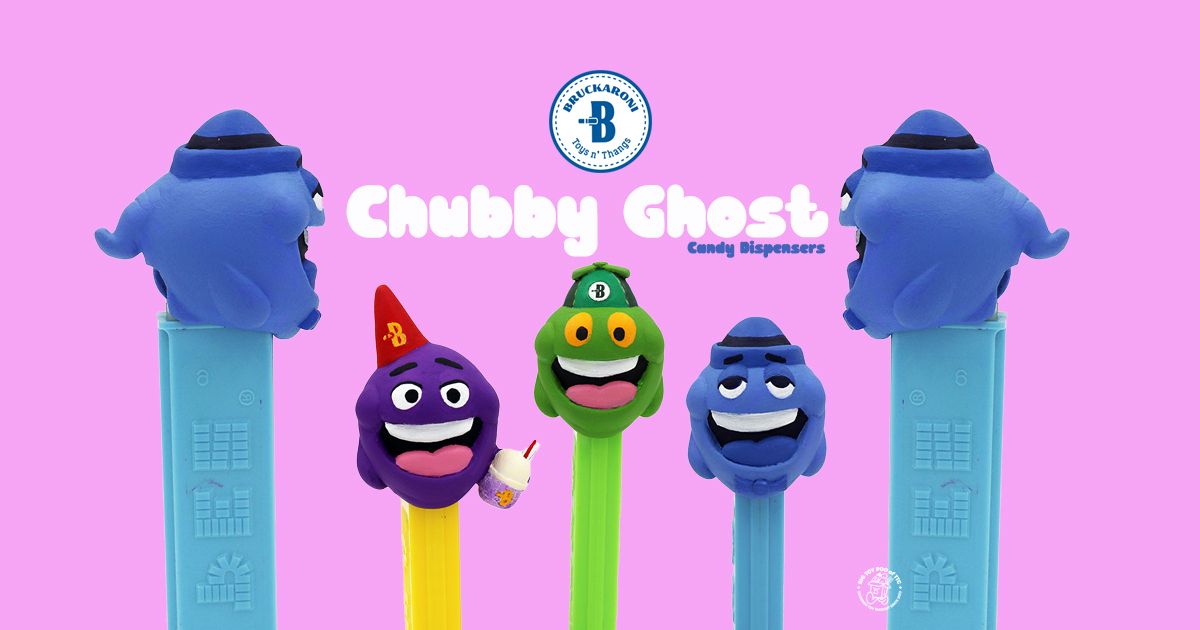This advertisement for "Chubby Ghost" PEZ dispensers features a vibrant pink background showcasing five candy dispensers. The leftmost and rightmost dispensers are blue, each adorned with a ghost-like character sporting white eyes with black pupils, small dark blue top hats with black stripes, and wide-open mouths, creating a friendly rather than scary appearance. These ghosts, sitting on cyan dispensers, are positioned towards the center and appear to gaze at one another.

In the center of the poster, a white circular logo outlined in blue dots, featuring a blue capital "B" and the company name "Bruckeroni," presides above the bold, white bubble-font text that reads "Chubby Ghost," with "Candy Dispensers" in a smaller blue font below it.

Three more PEZ dispensers lie below the text. From left to right: the first displays a smiling purple ghost with exposed upper teeth, a pink tongue, and a red party hat adorned with a "B." This character, holding a cup of what appears to be vanilla ice cream, is perched on a yellow dispenser. The second dispenser, light green, supports a green-faced ghost with yellow eyes, an open mouth, and a small green hat with a bee illustration. The third dispenser, similar to the bookend ones, is blue with a cyan base, featuring an identical ghost face and hat design. The entire arrangement highlights the joyful and playful design of the Chubby Ghost candy dispensers, making this a captivating and detailed advertisement.